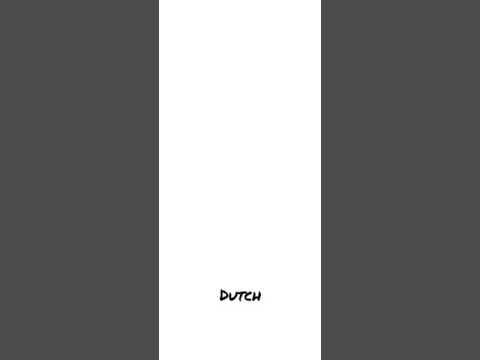The image is a square graphic, divided evenly into three vertical rectangular sections. The left and right sections are solid dark grey bars, while the middle section is stark white with no borders, seamlessly blending into the grey bars on either side. Near the bottom of the white center section, in small, black, all-caps font with a brush effect, the word "DUTCH" is prominently displayed. The overall design is minimalistic, featuring no other colors, shading, or additional imagery, which might suggest a modern or abstract representation potentially inspired by the Dutch flag in a monochrome style.